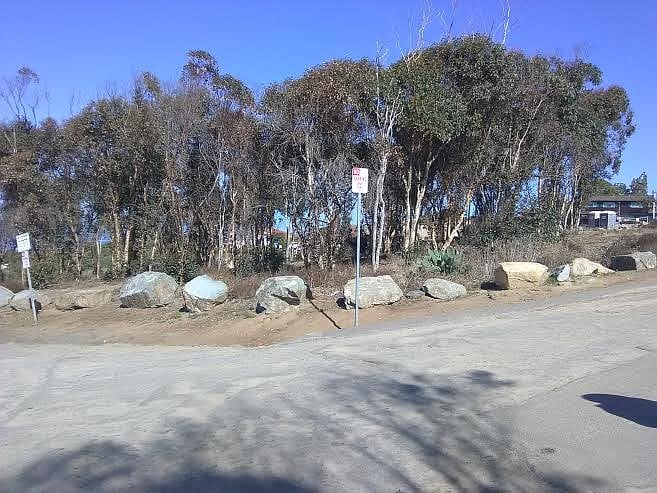The image captures a scene of an uneven, gray concrete roadway extending through the foreground. The road, devoid of markings, is accompanied by shadows of a person and trees, indicating broad daylight under a clear, blue sky. Alongside the roadway, a structure composed of large boulders serves as a protective barrier preventing vehicles from veering off into the adjacent terrain. The boulders rest upon brown dirt, accentuating the rough, natural setting. Mid-image, two signs stand out — a central, prominent "no parking" sign and a smaller, unreadable sign to the left. Beyond the rocky barrier, a dense line of thin-trunked deciduous trees with sparse, greenish-gray leaves extends into the distance. To the far right, partially obscured, a distant house emerges among the trees, adding a touch of human habitation to the scenic landscape.